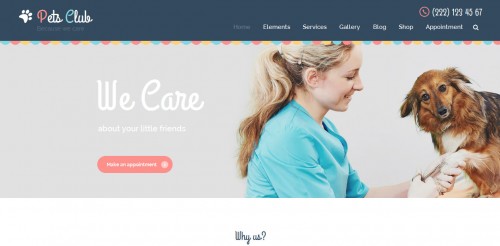The image features a visually engaging layout, beginning with a section in cursive writing accompanied by three distinct logos to the left: a white paw print, a symbol resembling a purple "P," and a white design. These elements introduce seven small categories, with the current selection highlighted in gray while the others are displayed in white. In the top right corner, there's a contact phone number. Below it, a light gray background displays the phrase "We Care" in cursive writing. 

A prominently placed reddish-pink oval button with white text adds emphasis to the layout. At the very top, the design is enhanced by a series of alternating yellow and light blue small circles. To the right, a side-view image of a woman with blonde hair in a ponytail, wearing a light blue shirt, is visible. She holds the paw of a brown dog that looks directly at the camera. Near the bottom center of the image, the phrase "Why Us?" is rendered in cursive on a white background.